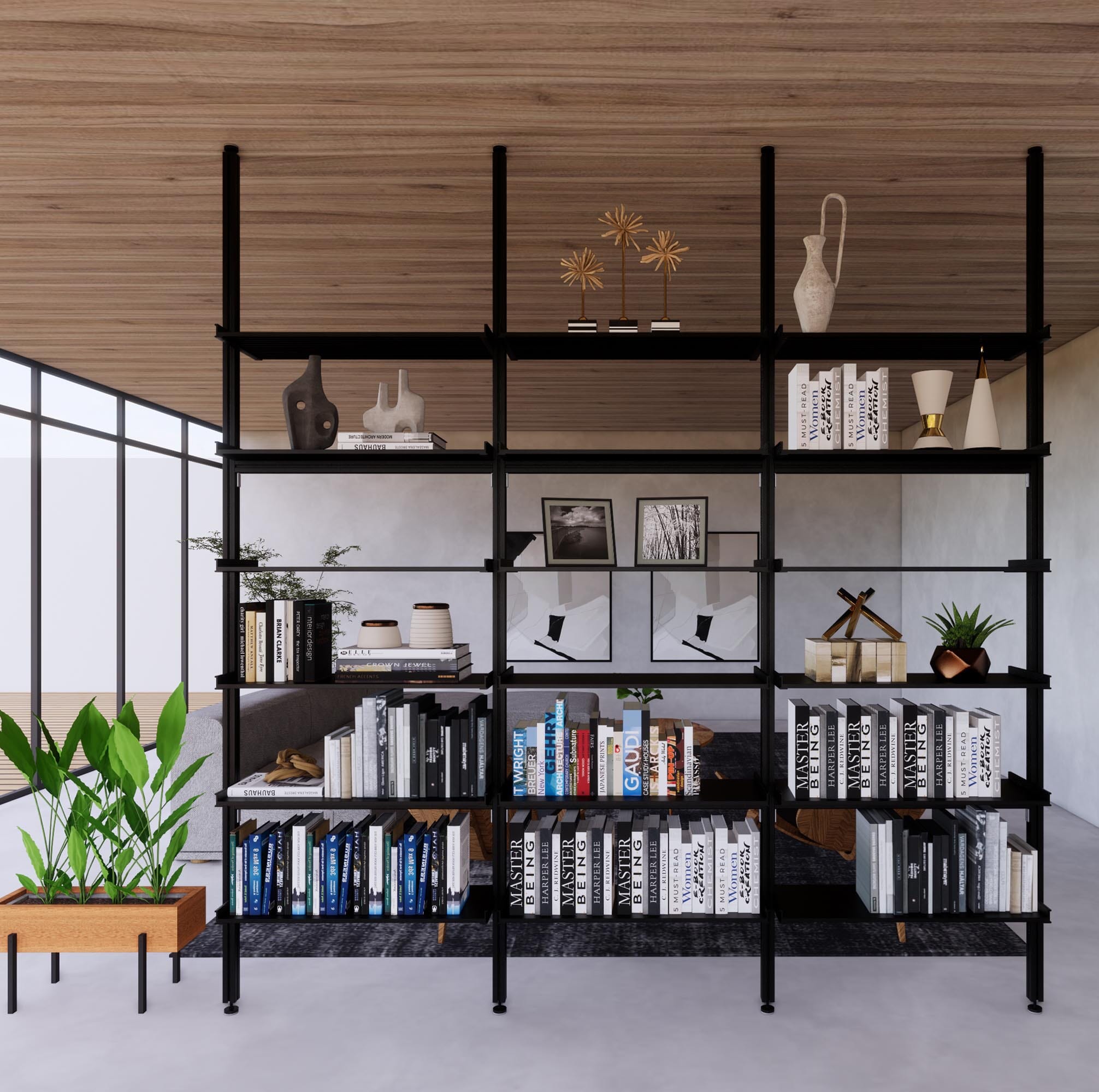This is a computer-generated artwork depicting a tall, black metal bookcase with six shelves, spanning from floor to ceiling, situated in a modern living room. The bookcase, organized into three bays, has the bottom two shelves filled with books. The middle shelf contains a combination of books and potted plants, while the next shelf up includes photographs and various decorative items. The top two shelves showcase ornaments, including vases and artistic decorations. A rectangular wooden planter with green plants sits on the floor to the left of the bookcase, next to expansive floor-to-ceiling metal-framed windows that let in natural light. The room features a wooden ceiling, gray concrete floors, and white concrete walls adorned with abstract art pieces. In the background, a couch can be seen, adding to the modern aesthetic of the space.